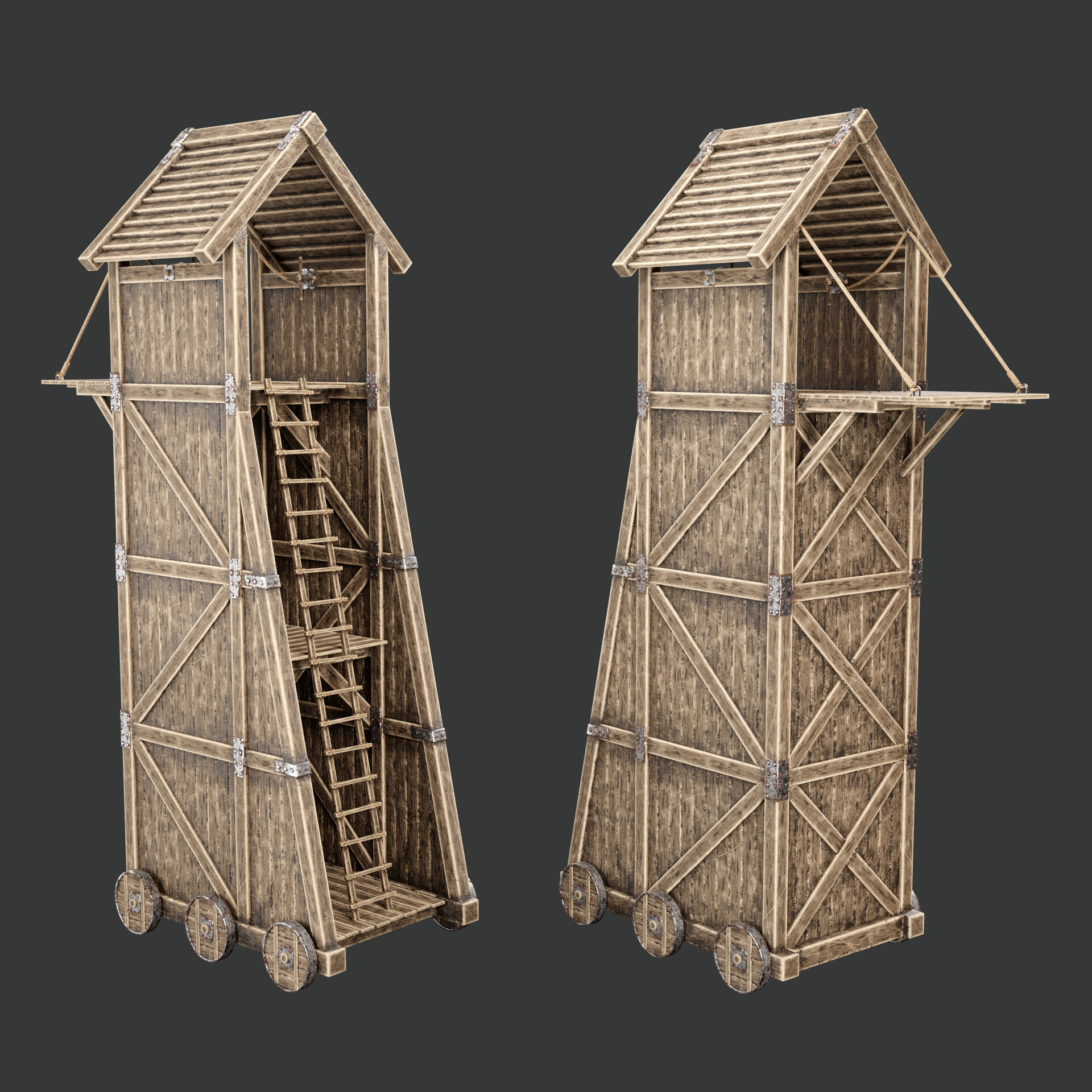The image depicts detailed illustrations of a medieval siege tower, displayed against a dark grey background. The wooden towers stand three stories high and are supported by six wooden wheels. Each tower features a sloped, traditional-style roof that helps to deflect attack substances such as oil. The image provides both front and rear views of the tower, showcasing its comprehensive design. 

The rear view reveals the internal structure with a ladder that allows soldiers to ascend from the bottom to the top. A wooden drawbridge, suspended by ropes or chains, is visible on the side, ready to be lowered when the tower is positioned against a fortress wall. Metal plating reinforces the corners, and wooden support struts criss-cross the panels for added stability. The front view shows the tower with its drawbridge down and the intricate detailing of the interior winch mechanism that operates it, as well as the structure of the wheels and the wooden panels. The careful portrayal of various angles and components enhances the understanding of this formidable piece of medieval warfare engineering.